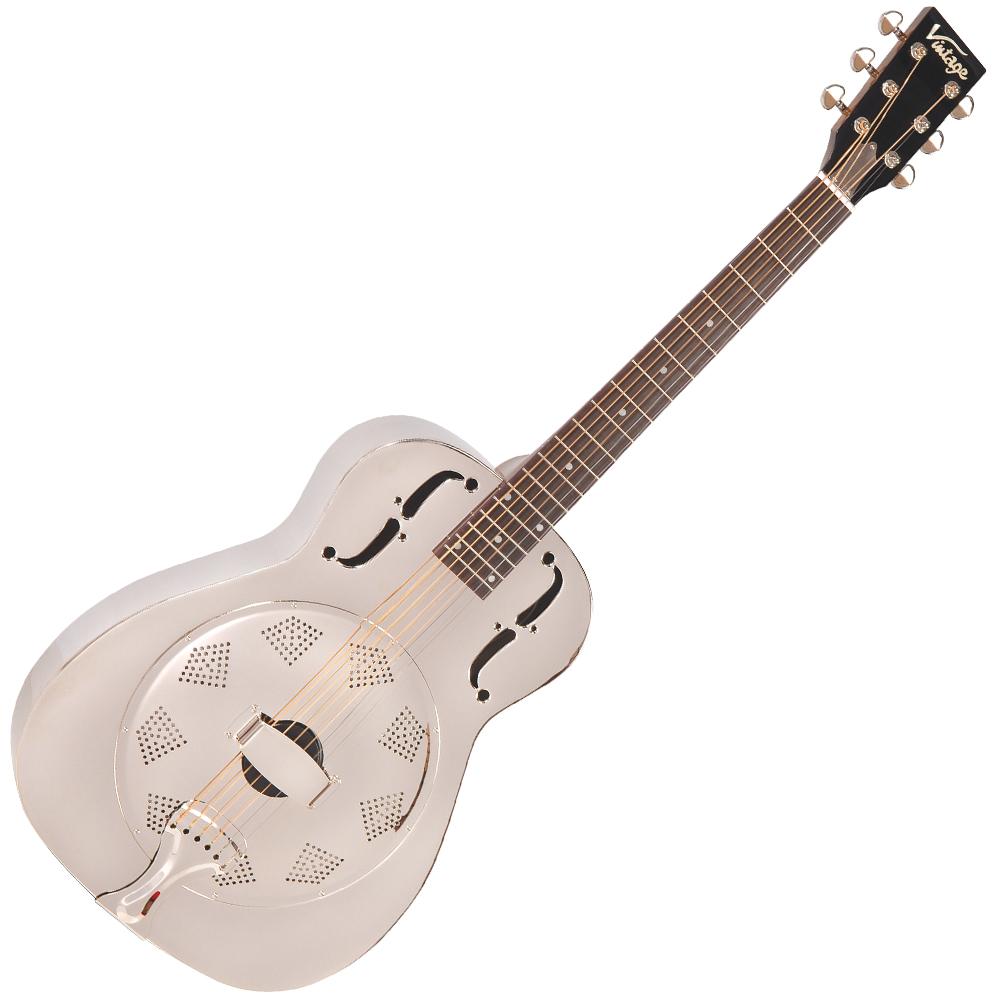The image depicts a vintage six-string banjo positioned diagonally against a pristine white background. The instrument's neck is a rich brown adorned with white horizontal line segments, and the headstock above it is black, featuring three silver tuning pegs on each side. Intricate details include shiny notches and gold or silver strings that glisten against their surroundings.

Centered on the pure white body of the banjo is a prominent circular metal plate with a hole in its center, framed by a rectangular white component. Elegantly contrasting this pristine background are two black S-shaped designs: a regular 'S' on the left side and an inverted 'S' on the right. Above it, on a black background, the word "vintage" is clearly inscribed in white. The overall aesthetic blends the rustic charm of the brown neck and black headstock with the meticulous elegance of the white body and golden elements, capturing both the visual appeal and the musical heritage of the banjo.